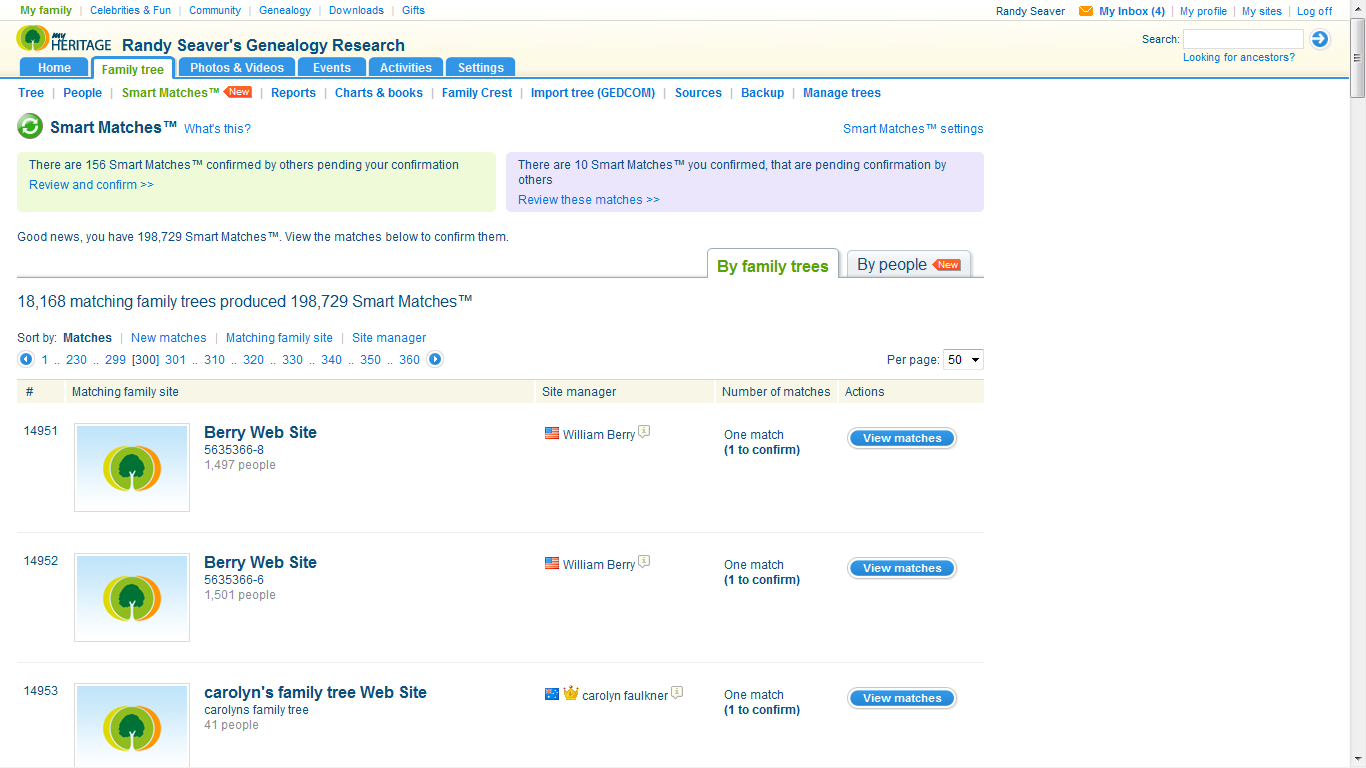The website "Heritage by Randy Sievers Genealogy Research" features an extensive and detailed family history exploration tool. The top navigation includes tabs for 'Family', 'Celebrities & Fun', 'Community', 'Genealogy', 'Downloads', and 'Office'. The text appears in very small font. On the right-hand side, there's a search bar for quick access.

Below the main navigation, additional tabs are organized into categories: 'Home', 'Family Tree', 'Photos & Videos', 'Events', 'Activities', and 'Settings'. Most of these categories are highlighted in blue, except for 'Smart Matches', which stands out in green and bold black lettering. Hovering over 'Smart Matches' brings up an informative tooltip explaining its function. 

A notification box reveals the current status of your Smart Matches: 155 matches have been confirmed by others and are pending your validation, and there are 10 matches that you have confirmed that are awaiting validation from others. The interface indicates an impressive total of 196,729 Smart Matches, which can be viewed and confirmed by filtering through family trees and individual profiles.

The tool essentially pulls in relative matches and provides direct links to access detailed family trees, allowing users to explore and confirm their genealogical history with precision.